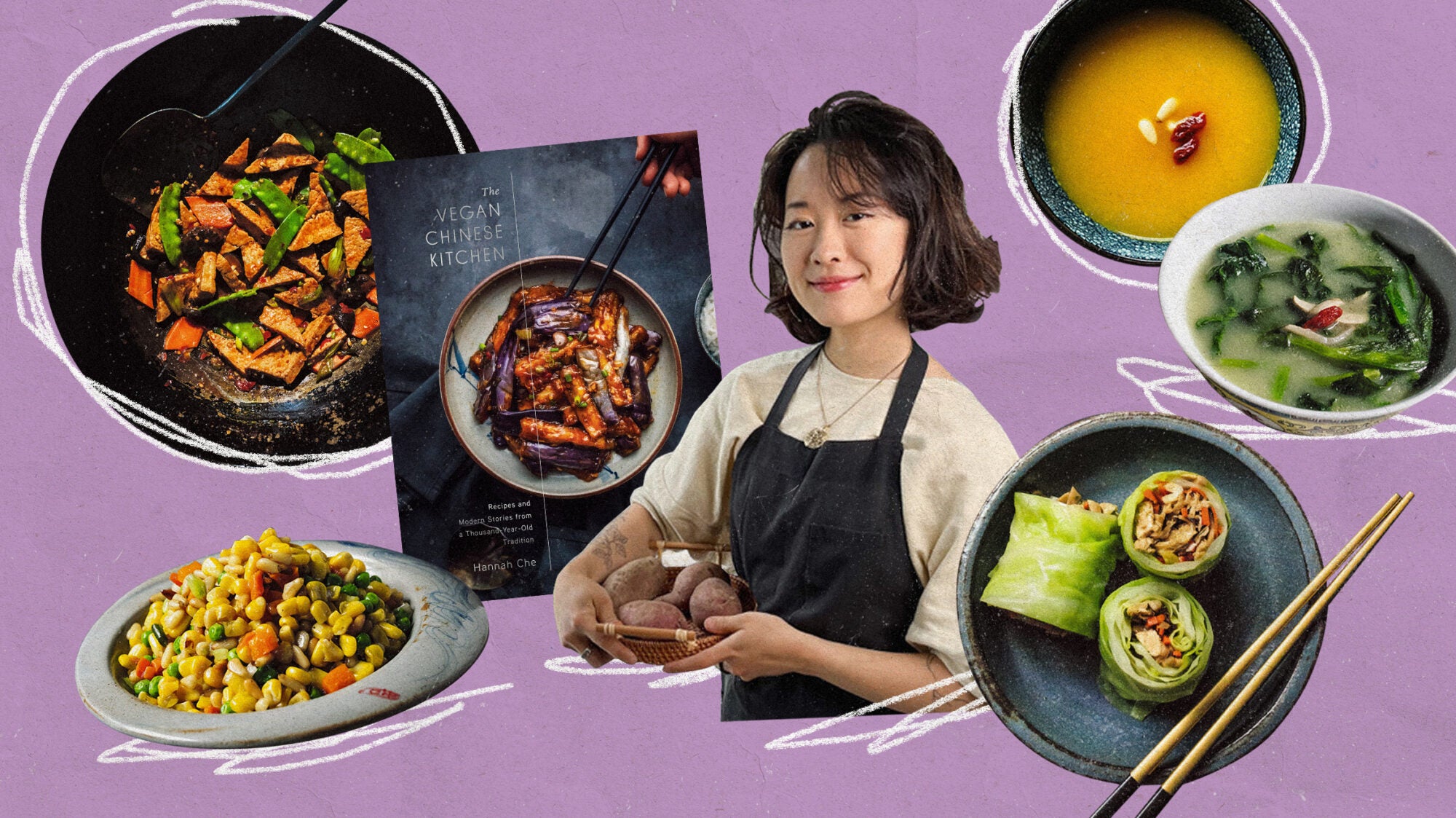The photograph features an Asian woman at the center, smiling and posing in a cream-colored shirt, black apron, and a necklace while holding a bowl of potatoes. She stands against a purple-pink background. Surrounding her is an array of vegan Chinese dishes and a cookbook titled "The Vegan Chinese Kitchen." To her left, the cookbook's cover is displayed, showing food in a pan with chopsticks. Below the book are two overlapping plates; the upper black plate contains a spoon, some greens, and food, while the lower white plate is filled with corn, tomatoes, and peas. In the bottom right corner, another black bowl holds salad wraps and chopsticks. The top right corner showcases two bowls of soups—an orange-based soup on top and a green-based soup below. Additionally, there is a paper underneath a frying pan near her.